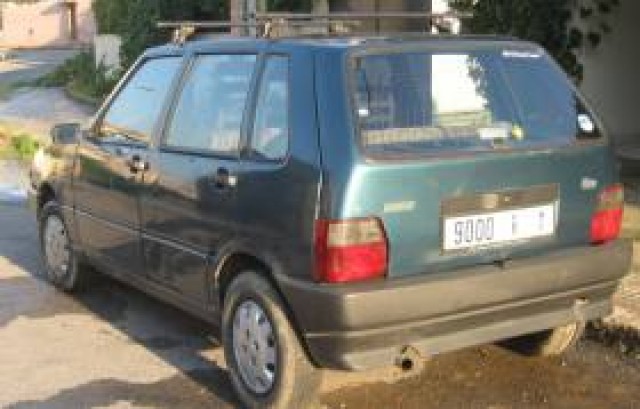The image captures the back and side of an older, darker green station wagon, prominently positioned slightly off-center towards the right. The vehicle features a luggage rack on top but is notably empty. You can faintly make out part of its white rectangular license plate, which appears to have the number '9000,' though the rest of it is blurred. The vehicle, characterized by its two doors, large back windshield, and a series of windows on the driver's side including a small triangular one, is parked on a road that appears wet, suggesting recent rain. The tires are worn and muddy, indicating heavy use. Surrounding the car, you can see the curb and some grass poking through the concrete road, with additional details like a stone walkway and a garage with a white door in the background. The scene is set in an outdoor residential area with distant houses or buildings, adding to the overall sense of the environment.